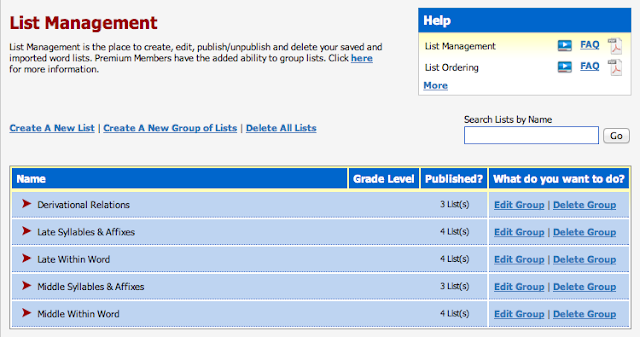Here's the cleaned-up and detailed caption for the image of the website:

---

The image depicts a website interface dedicated to list management. In the upper left corner, a maroon-colored heading reads "List Management." Below this heading, a description explains that "List Management" is the place to create, edit, publish, unpublish, and delete saved and imported word lists. For Premium members, there's an added feature to group lists. A clickable link in blue text says "Click here for more information."

In the upper right corner, there's a section for help, marked by a blue box with white text that says "Help." This section provides a list of FAQs and videos for guidance on list management. It includes similar support for list ordering, with both FAQs and instructional videos available. Additional options are noted in blue text with an underline.

The central part of the website body features user actions such as "Create a new list," "Create a new group of lists," or "Delete all lists." Adjacent to these options, a search bar allows users to search lists by name, accompanied by a "Go" button to initiate the search.

In the lower part of the website, a blue box with a yellow outline lists categories and options. The categories include "Name," "Grade Level," "Publish?" and "What do you want to do?" Listed examples of word lists include "Derivational Relations," "Late Syllables and Affixes," "Late Within Word," "Middle Syllables and Affixes," and "Middle Within Word." Each listing shows the number of lists available and provides options to edit the group or delete it.